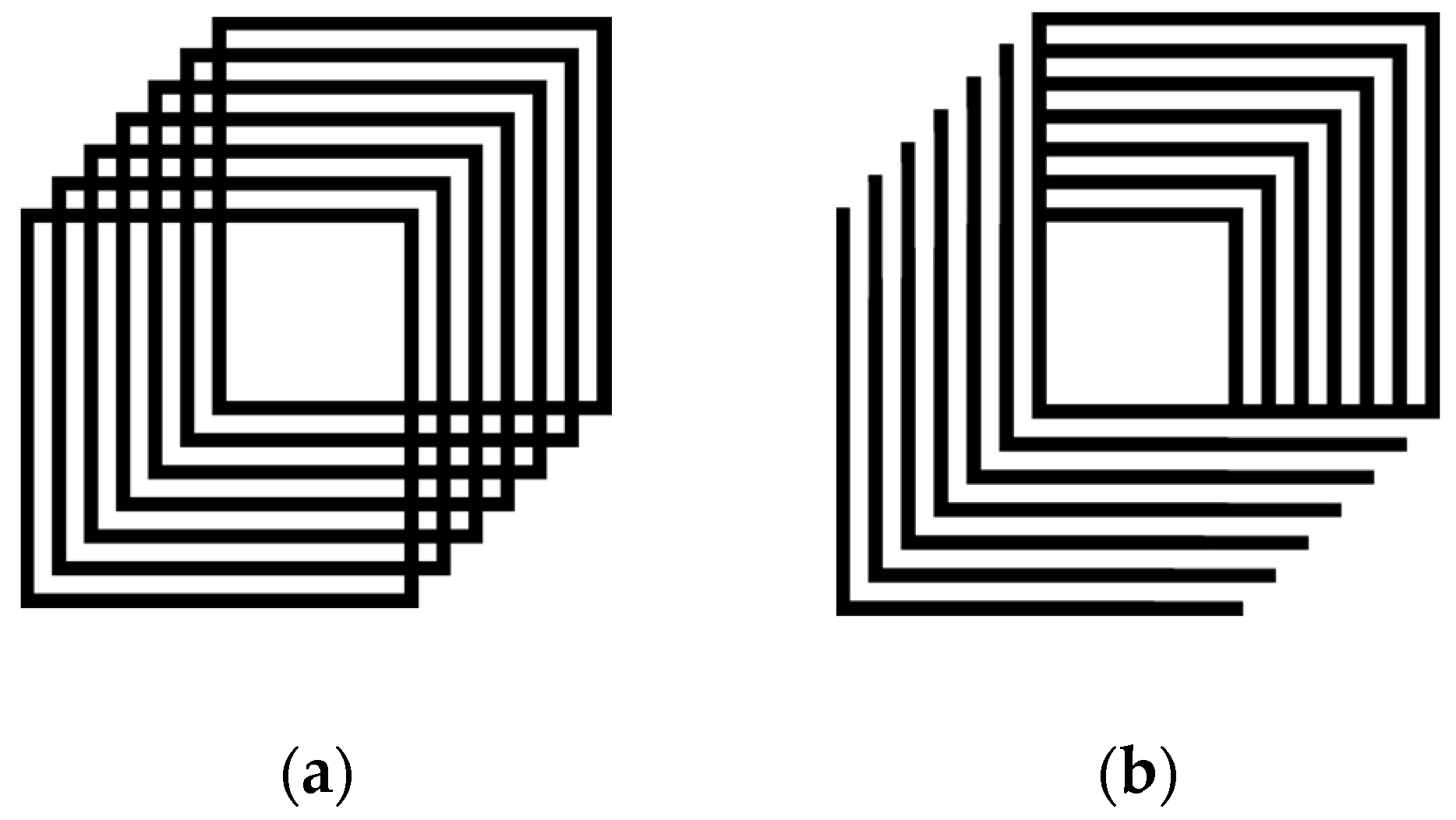The image displays two geometric diagrams on a white background. On the left, labeled with (a), there is a schematic representation comprising seven black-outlined squares. These squares create a tunnel-like illusion due to their staggered alignment: the front square is positioned slightly to the left, and each subsequent square shifts gradually to the right. This arrangement yields a visual effect where the squares appear to recede into depth.

On the right side, labeled with (b), there is an alternative design also featuring seven black-outlined squares. In this configuration, the squares form an inverted pattern compared to the left. The initial square is positioned at the top, with each subsequent square descending diagonally. Unlike the consistent square outlines of the left diagram, only the outer edges of the squares are drawn, giving the appearance of incomplete or detached "L" shapes. This creates an impression of a more open, descending tunnel effect.